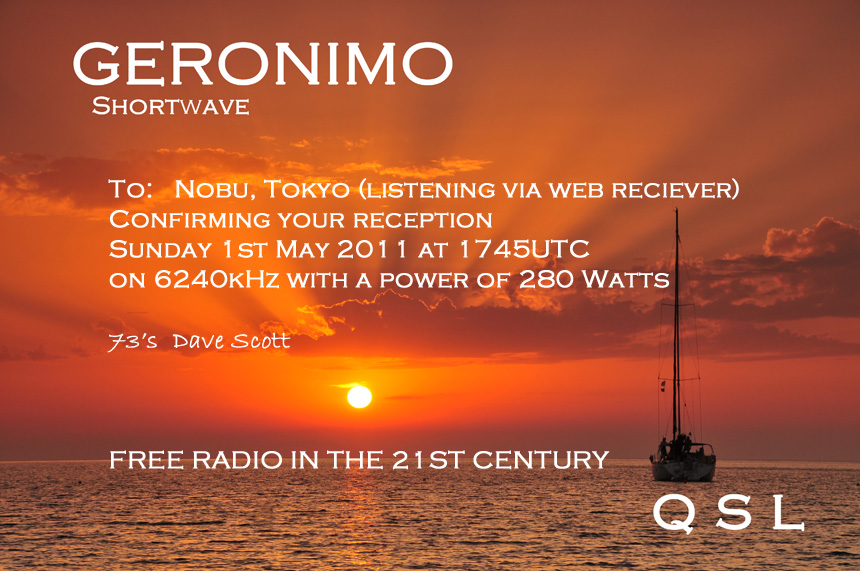The image features a serene photo of calm ocean waters taken at sunset. The sky, painted in vibrant orange hues, is adorned with scattered clouds and the glowing sun positioned just above the horizon. A silhouette of a sailboat without sails is floating on the water to the right. Overlaying this tranquil scene is a heading in white capital letters at the top left corner: "GERONIMO A SHORTWAVE." Beneath it, also in white capital letters, the text reads: "To Nobu Tokyo, listening via web receiver. Confirming your reception Sunday 1st May 2011 at 1745 UTC on 6240 KHz with a power of 280 watts. 73's, Dave Scott. Free Radio in the 21st Century." In larger white letters, the abbreviation "QSL" appears towards the bottom right of the image. The overall design integrates the white text seamlessly with the sunset background, providing a visually appealing and informative depiction.